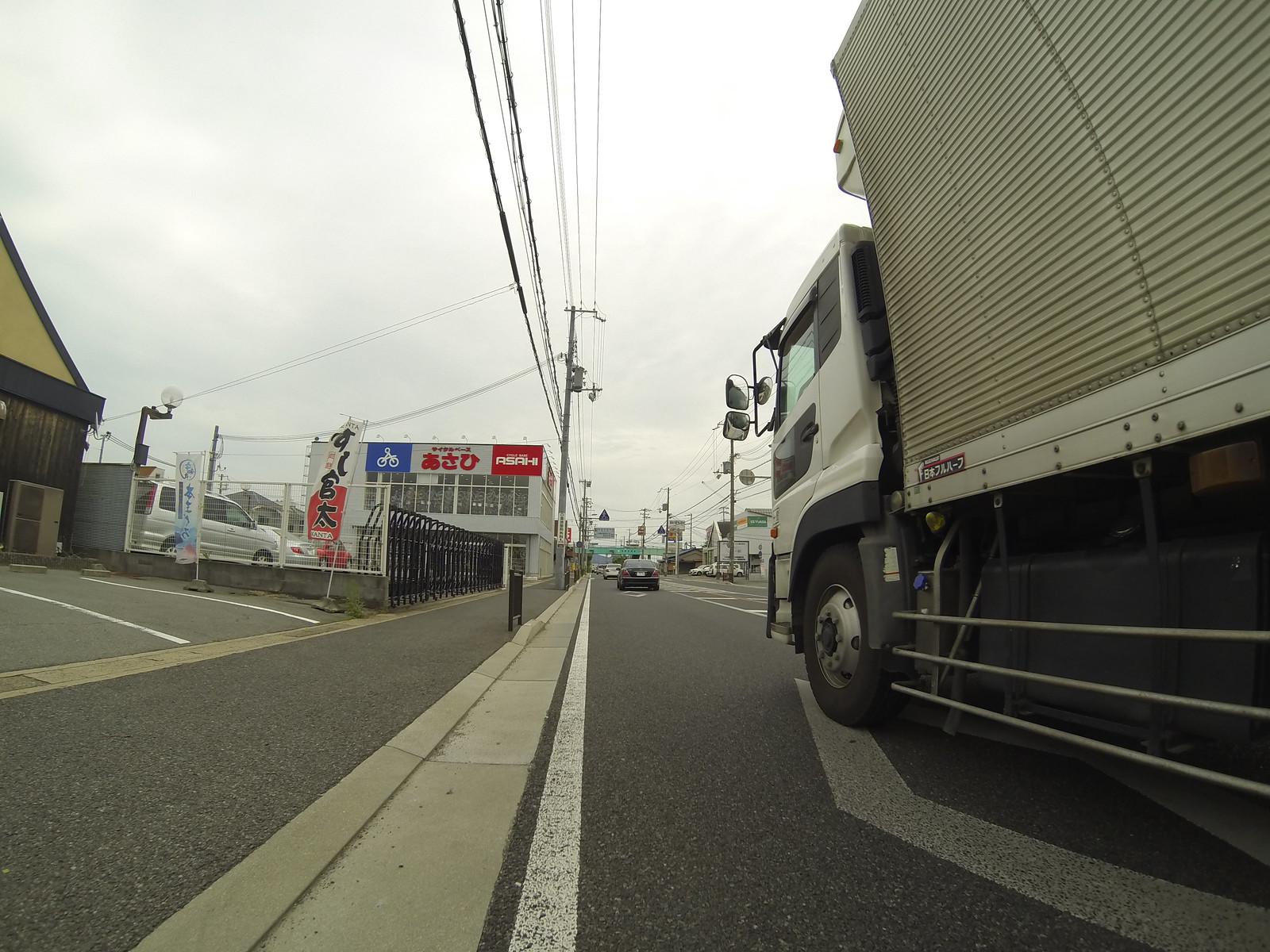The image depicts a bustling street scene from a vantage point close to the ground, angled slightly upward, capturing a wide view of an international urban setting. On the left side of the road, a parking lot is visible, filled with several cars, and adorned with signage presumably guiding vehicles to designated parking spots. The surrounding buildings and banners feature text in a foreign language, indicative of the image being from another country. The street itself is lively with multiple cars driving down the road. Prominent power lines stretch across the scene, and a large truck, possibly a semi-trailer though not definitively an 18-wheeler, can be seen carrying a load. The road markings include lines and diamond shapes, the specific meanings of which are unclear. Overall, the street appears very busy, contributing to the dynamic and energetic atmosphere captured by the photograph.